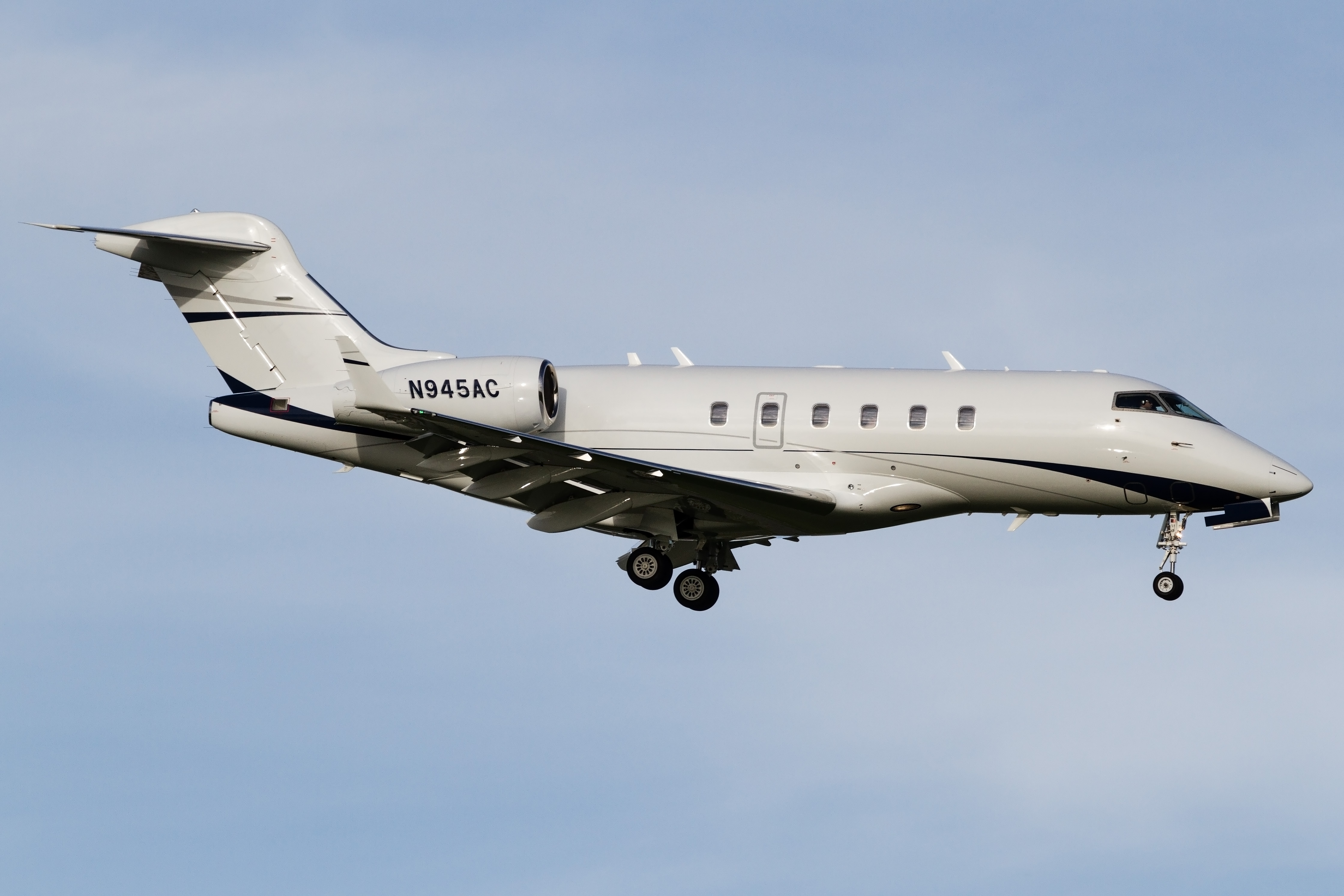The photograph captures a sleek, aerodynamic jet engine plane flying to the right, prominently displayed in the center of the image against a light blue sky. The plane's white body is accentuated by black stripes running from its pointed nose to the rear. Its landing gear is fully extended, with all three black wheels visible. The plane has a distinct registration on its engine that reads "N945AC." Along the fuselage, there are five windows and a door with an additional window. The cockpit reveals a pilot looking towards the bottom left. The plane also features three fin-like structures on its top rear. The overall appearance suggests the plane is in the process of landing.